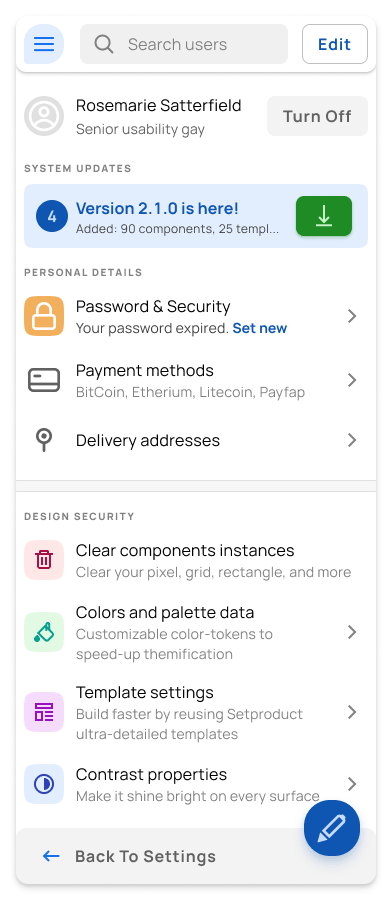The image showcases a user interface of an application predominantly in a white theme with accents of blue, green, orange, red, purple, and black fonts. At the top, there's a gray search bar featuring a magnifying glass icon and the placeholder text "Search Users." To the right of the search bar is a blue "Edit" button. 

Below the search bar is a gray circle profile button next to the name "Rosemary Satterfield" with an option labeled "Turn Off." Rosemary Satterfield is identified as a "Senior Usability Gay." 

The interface includes a section for system updates, highlighted by a blue bar with a blue circular icon labeled "4." In blue font, it indicates "Version 2.1.0 is here." There is a green download button with a download arrow and the text "Add an ID components with 25 templates."

Further down, there is a section titled "Personal Details," featuring an orange square box with a white lock icon labeled "Password and Security." Other options visible are a payment method icon representing a credit card and delivery addresses indicated with a pin icon. 

Additionally, there's a red box with a trash can icon for "Clear component instances," and a section for "Colors and Palette Data."

This detailed depiction helps users navigate and understand the functionalities provided within the application.